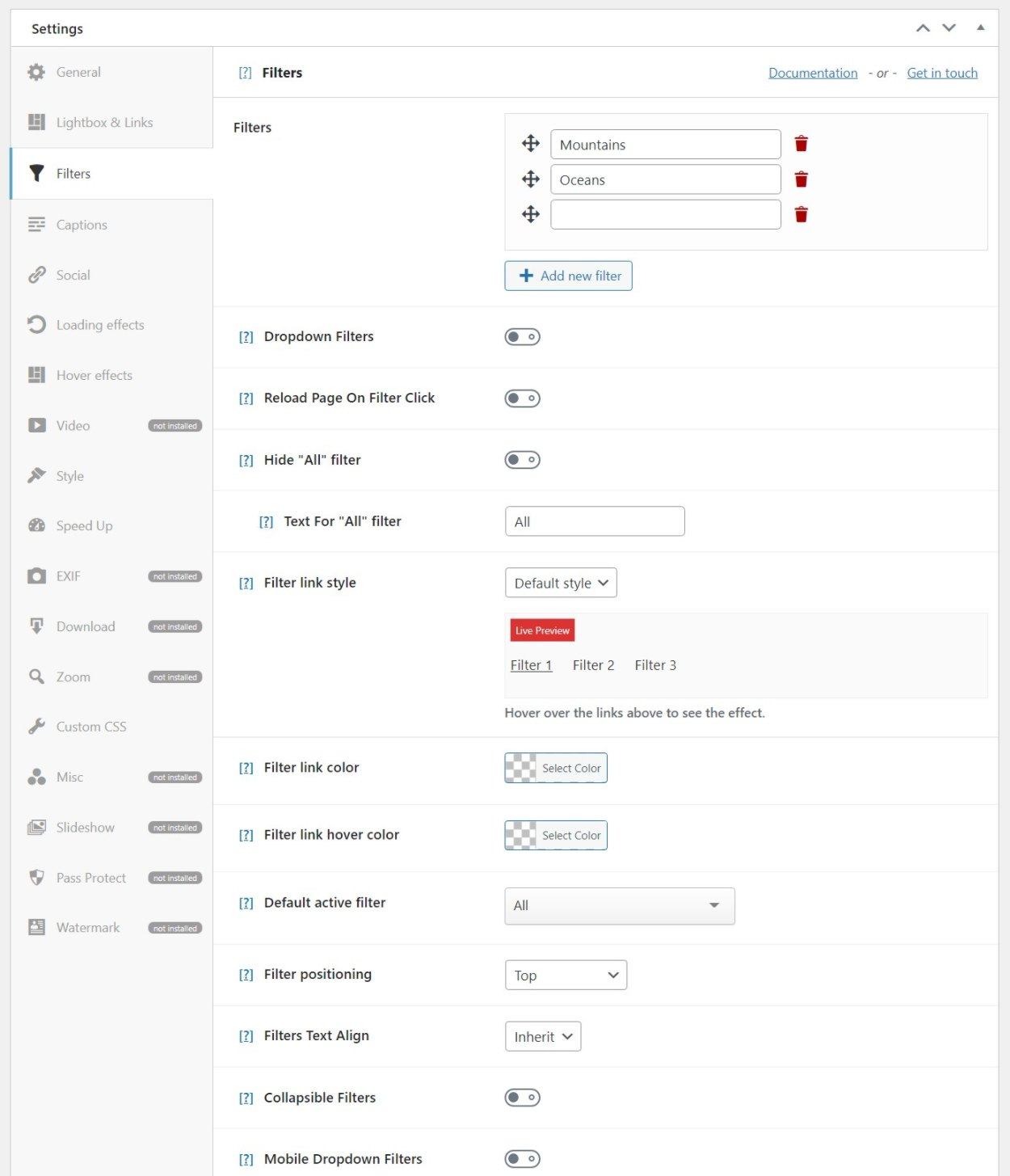**Detailed Descriptive Caption:**

The image depicts a tall, vertically oriented settings page on a laptop screen. The bottom section of the image is cut off, and the entire content area is bordered in gray. 

At the top, there is a long white bar with the word "Settings" displayed in black in the upper left corner, while on the far right, there is a vertical black V-shaped icon. Adjacent to this is a gray menu bar on the right side, featuring various clickable icons. Recognizable icons include a magnifying glass labeled "Zoom" in gray text, a wrench, and a refresh icon. Beside each icon, small gray text describes their function, although the text is quite difficult to read. Notably, the third icon down is clicked and highlighted, displaying the word "Filters."

Below the main settings header, there's another long white bar containing a small gray icon to the left and the word "Filters" in black to the right. On the far right side of this bar are underlined, hyperlinked terms "Documentation" and "Get in Touch" in gray.

Further down, there is a section titled "Filters" again, which features three text boxes for user input. The first box contains the word "Mountains," the second "Oceans," and the third is blank. Next to each text box is a red trash can icon for deletion.

In the central part of the settings page, several options are delineated by thin gray lines. Each option is prefixed by a question mark icon, followed by drop-down filter options. Key options listed include "Reload page on filter click," "Hide all filters," "Test for all filters," and "Filter link style." To the right of the top three options are toggle switches with gray circles positioned to the left, indicating an off position.

Beneath these options is a red box with white letters that are too small to discern. Below this red box, filters are sequentially labeled “Filter 1,” “Filter 2,” and “Filter 3,” shown as highlighted boxes. Below this area, in gray text, it states: "Hover over links above to see the effect," though the text is somewhat hard to read. A thin gray bar is present below this instruction.

Further down the settings page, additional options are shown from top to bottom, including "Filter link color," "Filter link hover color," "Default active filter," "Filter positioning," "Filter text align," "Collapsible filters," and "Mobile drop-down filters." To the right of the top two options is a gray and white checkered box within a gray area, labeled "Select color."

Below this checkered box is a drop-down menu labeled "All," followed by another drop-down menu at the bottom labeled "Top." Another drop-down menu, which says "Inherit" in black text, is positioned beneath that. The final two options on the right side each have a toggle switch, both toggled to the left with gray circles indicating an off position.